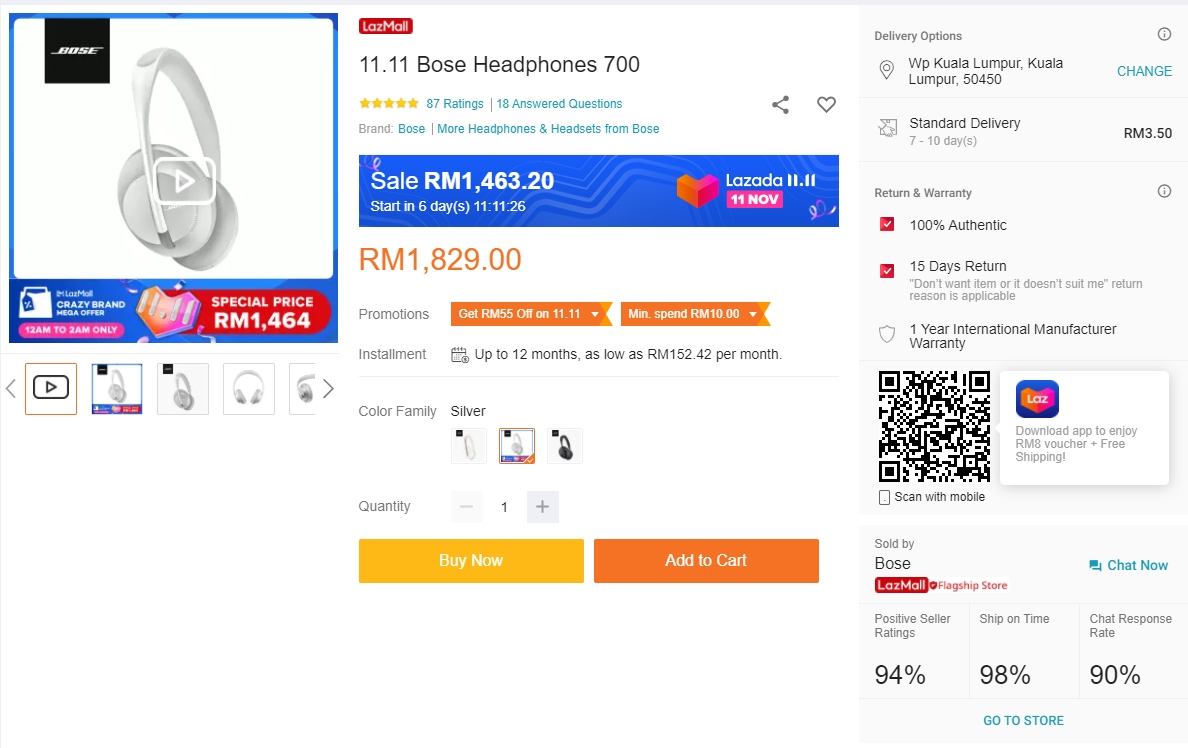Screenshot of an anonymous shopping website displaying the contents of a shopping cart. The cart contains a pair of Bose 700 headphones priced at RM 1,829, where 'RM' stands for Malaysian Ringgit. The user interface includes a prominent yellow "Buy Now" button and an orange "Add to Cart" button. To the right of these buttons, there are delivery options, specifying a shipping address in Kuala Lumpur, Malaysia, with an estimated standard delivery time of 7 to 10 days. No clear indication of the website's name is visible in the screenshot.